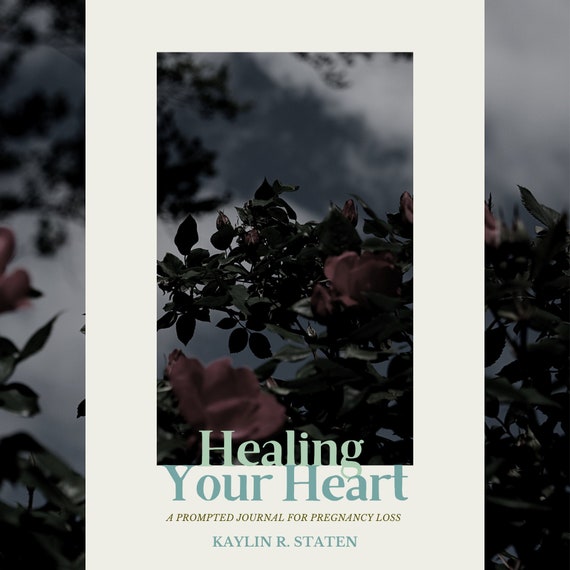The image is a three-part cover for a book titled "Healing Your Heart: A Prompted Journal for Pregnancy Loss" by Kaylin R. Statton. Set against a cream-colored background, the cover features a photo that is intricately sliced into narrow strips, creating a fragmented yet visually compelling design. The background of the photo appears to be taken outside, likely at night, with foggy conditions that lend a somber atmosphere. It showcases a rosebush with dark red flowers in the foreground, evoking a sense of broken beauty and poignant reflection. 

The photo is overlaid with a thick white border in the central portion, which captures branches and flowers, subtly hinting at growth and healing amidst loss. The title "Healing Your Heart" is prominently displayed in the middle section, with "Healing" in light green and "Your Heart" in teal. The subtitle is written in a tannish brown color, stating "A Prompted Journal for Pregnancy Loss." Below the subtitle, the author’s name, Kaylin R. Statton, appears in a light blue hue. The design of the sliced-up photo, combined with the delicate yet striking color scheme, powerfully conveys the book's theme of mending a broken heart.